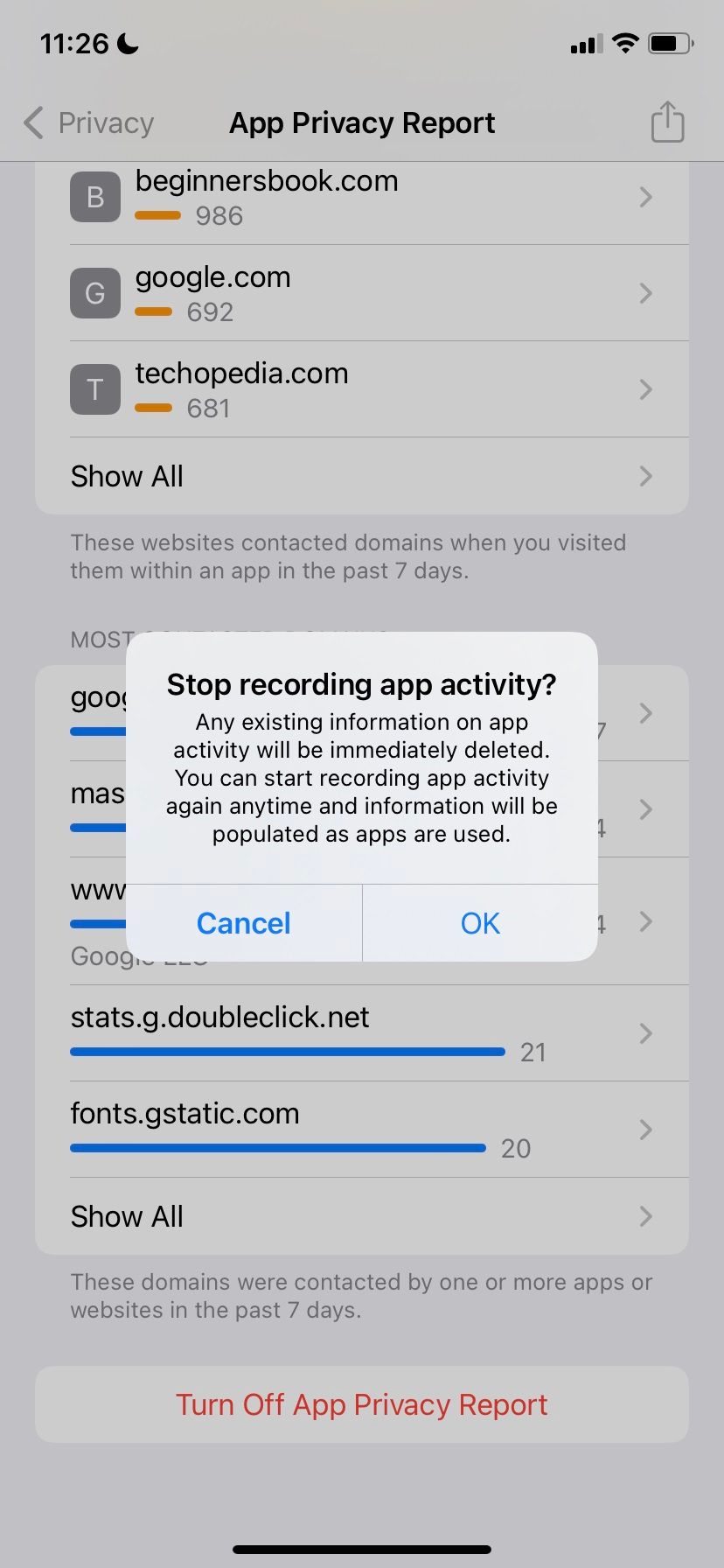The screenshot features a privacy report from an app, displaying an assortment of icons and data. 

At the top of the image, the status bar shows the time "11:26" in black text, alongside a crescent moon icon, indicating the device is in Do Not Disturb mode. On the right side of the status bar, there are standard icons for Wi-Fi signal strength, cellular signal strength, and battery level.

Beneath the status bar, the background is predominantly white but slightly grayed out due to the visibility of a pop-up message in the middle portion of the screen. The main content area of the screen starts with the heading "Privacy Report," accompanied by a box icon with an upward arrow within it.

Below the heading, there is a list of websites that have contacted domains when visited within an app over the past seven days:
1. "beginnersbook.com" is represented by a gray and white "B" icon and has a yellow line indicating "986" contacts.
2. "google.com" is marked with a gray "G" icon and shows "692" contacts.
3. "techopedia.com" has a gray "T" icon with "681" contacts.

An option to "Show All" is provided, along with a descriptive note stating, "These websites contacted domains when you visited them within an app in the past seven days."

The prominent pop-up message in the middle of the screen, displayed with black font on a white background, reads:
"Stop recording app activity. Any existing information on app activity will be immediately deleted. You can start recording app activity again anytime and information will be populated as apps are used."
Options to "Cancel" or "Okay" are presented in blue text.

Below the pop-up, there are additional boxes with black text and blue progress bars—partially obscured by the pop-up. The visible entries are:
1. "stats.g.doubleclick.net" with a blue bar indicating "21" contacts.
2. "fonts.gstatic.com" with a blue bar indicating "20" contacts.
An option to "Show All" in black text is also available.

At the bottom of the list, in gray text, it states, "These domains were contacted by one or more apps or websites in the past seven days." The screen concludes with an option in a red box reading "Turn Off App Privacy Report" and is bounded by a thin black line at the bottom.